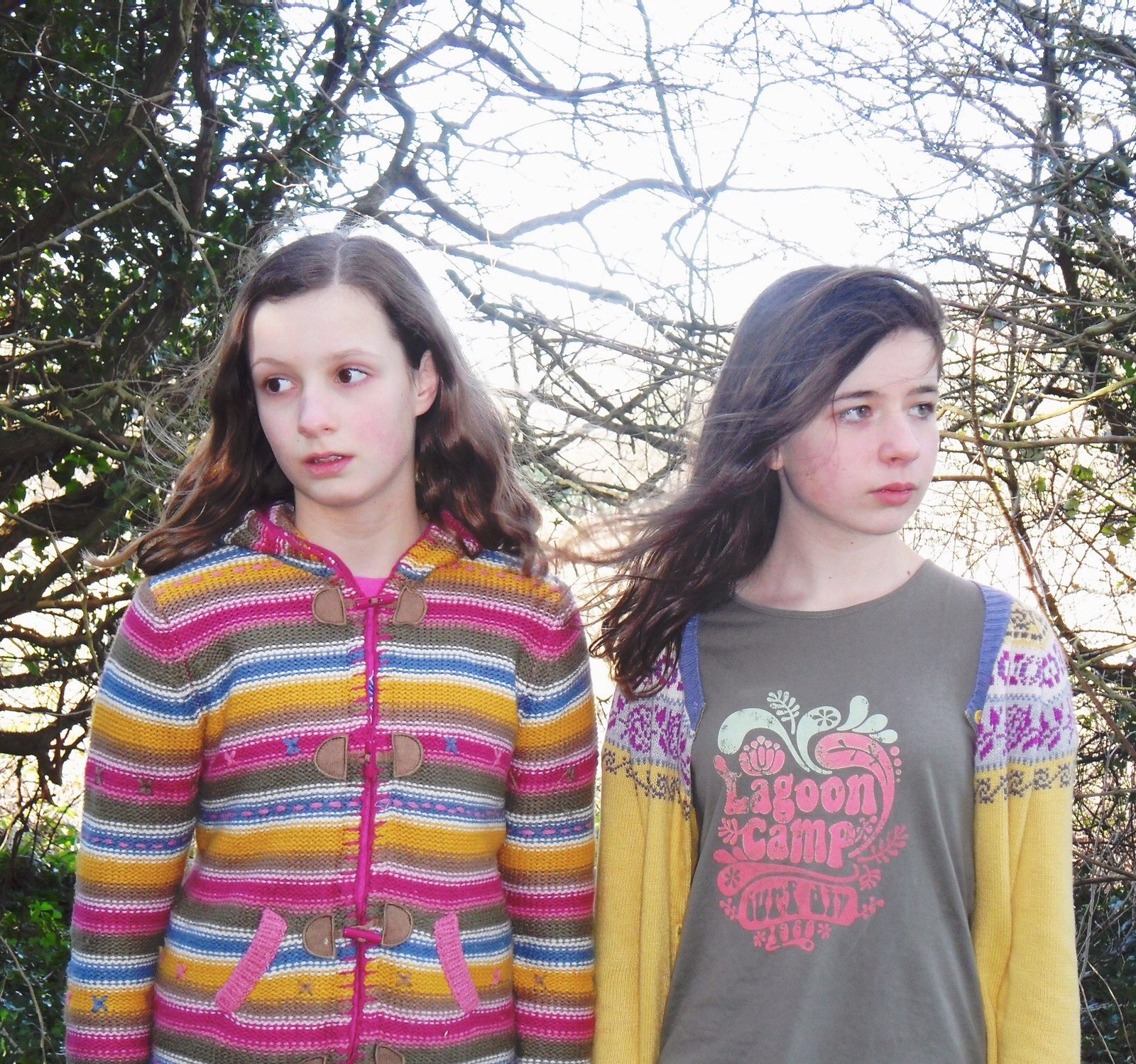In this picture, two young girls, approximately 12 to 13 years old, are standing side by side. Both are Caucasian with long brown hair and are looking away from each other—one to the right and the other to the left. The girl on the left is wearing a vibrant, multi-colored coat featuring stripes in yellow, orange, blue, pink, brown, gold, and white. Her coat has pockets and a hood. She has a slight grimace on her face and is wearing lipstick. Her companion on the right is wearing a greenish-brown t-shirt with the text "Lagoon Camp" printed in pink, embellished with decorative white flowers. Over her t-shirt, she has on a yellow coat. She, too, has a grimace and lipstick on her face. The backdrop consists of barren trees suggesting a fall or winter setting, with a white, overcast sky visible through the branches. Some sparse leaves are noticeable in the top left and bottom of the image.